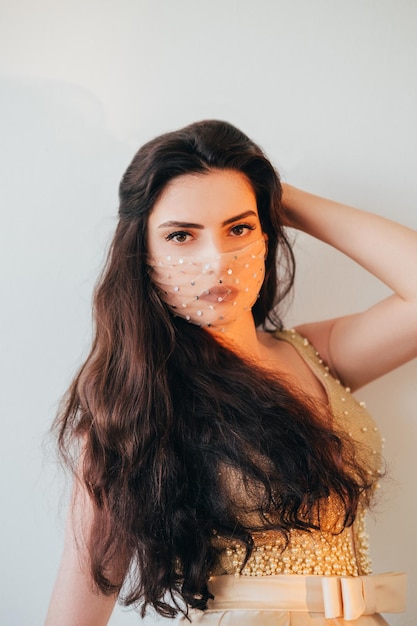The image depicts a beautiful brunette woman, possibly a belly dancer, standing against a white background. She has long, dark brown hair that cascades down to her waist and is swept over her right shoulder. Her striking brown eyes and dark eyebrows are visible above a clear veil adorned with golden studs, which covers the lower half of her face from her nose to her chin, allowing her red lips to peek through. She is posed with her left arm bent above her head, her hand resting behind it, and her right arm visible from the shoulder to the elbow.

The woman is wearing a gold dress with straps, decorated with white and gold studs. The top part of the dress is heavily beaded, transitioning to a cream-colored lower half. A tan belt cinches her waist, emphasizing the dress's ornamental design. She also has bare arms, adding to the detailed and exotic nature of her attire. The woman exudes a youthful and captivating presence, staring directly into the camera.